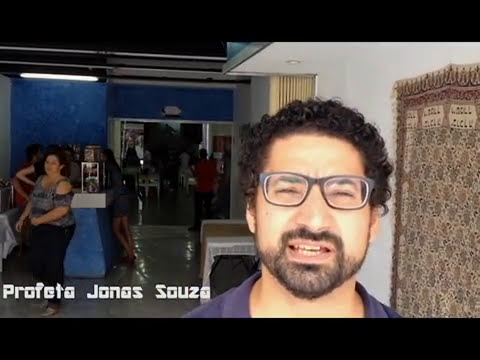In the foreground of this image, a young man with light brown skin dominates the right side, featuring black curly hair, short in length, and a neatly groomed black beard. He wears black-framed glasses, and his eyes are slightly squinting while his mouth is open, showing both his upper and lower teeth as if captured mid-sentence. His attire includes a dark blue shirt, visible primarily at the neckline. Positioned behind him is a white and blue room. To his immediate right, a textured rug or patterned poster featuring yellows with red circles and Arabic cursive writing at the top hangs against a white wall. In the bottom left corner of the image, white text reads, "Profeta Jonas Sousa."

Further back, the scene opens up to what appears to be a commercial area with a cafe-like stall, complete with cabinets and a countertop. Various people occupy this background: one young woman is walking off to the left, another is leaning against the counter engaging with people on the other side, and an elderly or middle-aged woman in a blue shirt and black trousers is also present. The scene is well-lit with a long, bright light shining down from the top left corner, illuminating the blue walls and the entryway leading to another indoor space, suggesting a bustling indoor environment potentially set in a commercial store or an area with cultural significance, possibly in the Middle East.